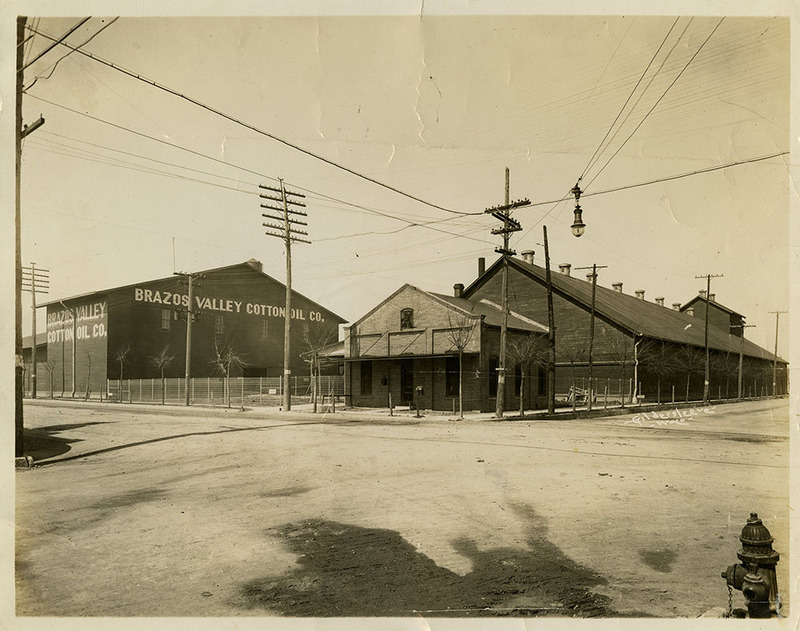This early 20th-century, black-and-white photograph captures a historical intersection featuring the Brazos Valley Cotton Oil Company, a notable manufacturer of its time. The scene is set at a crossroads, identifiable by the dirt roads and absence of stop signs, giving a clear view of the surrounding buildings. On the right side of the image stands a lengthy, one-story wooden building with an attic, while the left side features a taller, two-story structure that appears to be part of an industrial complex. Both structures prominently display the company's name in white text: "Brazos Valley Cotton Oil Company."

A lone, vintage street lamp and power lines crisscross above the road, suggesting an era when cable cars and telephone lines were common. The street below is unpaved, emphasizing the age of the photograph. In the bottom right corner, a distinctly visible fire hydrant stands with a slight wet patch around it. Additionally, large telephone poles equipped with substantial glass conductors indicate the technological infrastructure of the period. This photograph deeply immerses the viewer in the industrial and urban setting of the early 1900s.